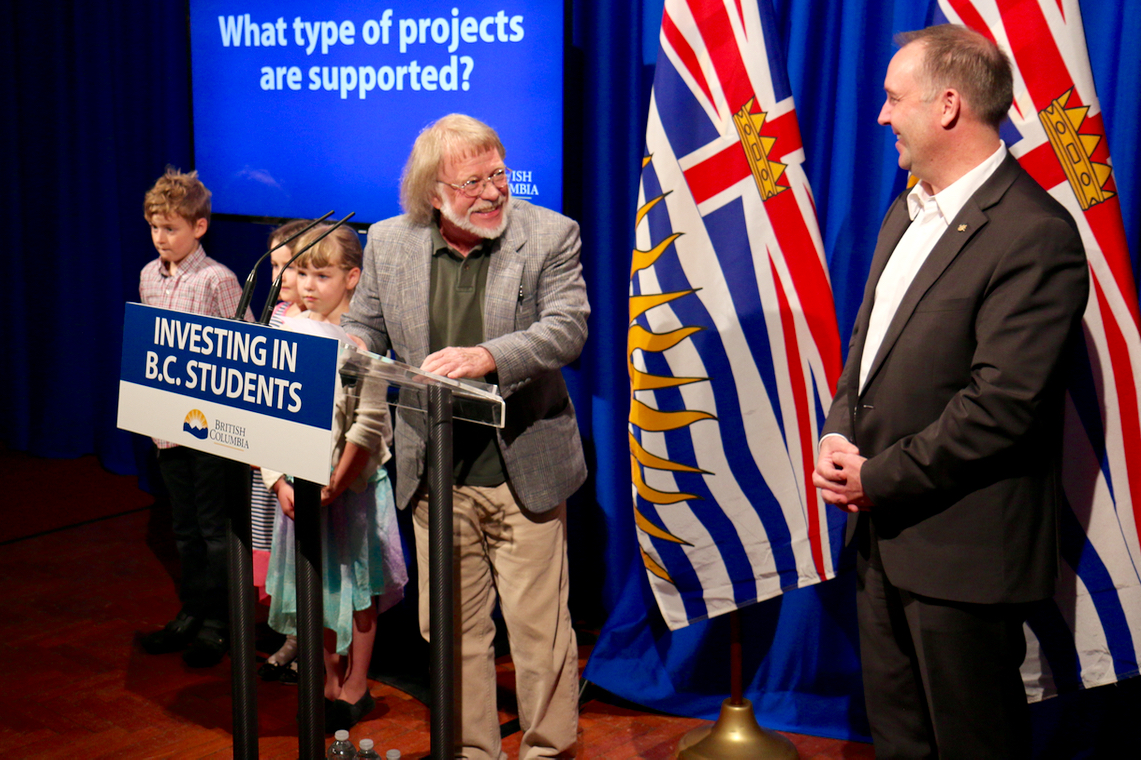A detailed scene unfolds on a school auditorium stage, featuring a diverse group of individuals centered around a podium. The background is dominated by a blue curtain and a TV screen displaying the text "What types of projects are supported?" in white letters. In front of the podium, a sign reads "Investing in BC students," set against the same blue backdrop.

At the podium stands an older gentleman, distinctive with shoulder-length blond hair, a gray stubbly beard, glasses, and a longer green polo shirt under a gray jacket paired with beige khaki pants. He exudes a professor-like aura. To his right, facing him, is a taller, younger man dressed in a brown suit with an open white collar, hands clasped and smiling courteously.

On the left side of the podium, three school-aged children stand slightly apprehensive but neatly dressed. The children consist of one young boy and two girls, all positioned prominently on the stage. In the background, flags featuring red, white, and blue with gold crowns and sun rays, likely symbols of British Columbia, add a ceremonial touch to the scene.